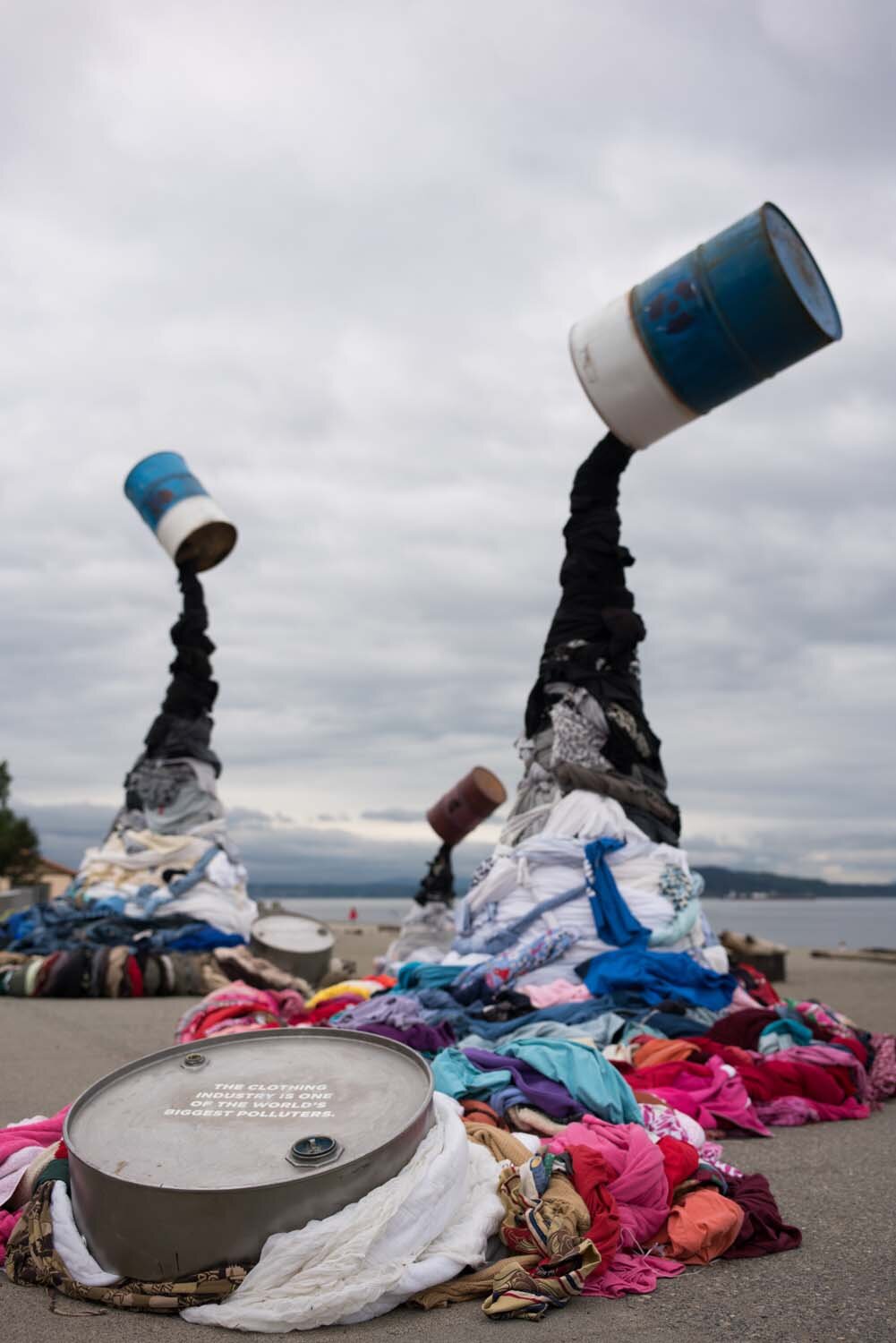This captivating outdoor photograph showcases a surreal and thought-provoking art installation set against a vast, gloomy seascape. In the background, a large, cream-colored body of water, likely an ocean, stretches out beneath an overcast, entirely cloud-covered sky, while distant hills fade into the horizon.

Dominating the sandy beach in the foreground stand two peculiar spires. Each spire features blue-and-white barrels, reminiscent of those used for burning trash, dramatically suspended in mid-air, side by side. Below these floating barrels, the artwork cascades into chaotic piles of clothes and plastic debris, evoking a sense of pollution and waste. Near the bottom of one spire, a smashed barrel lies amidst the mess.

One of the spires intriguingly includes an upside-down oil can, frozen in stasis as it pours out oil that elegantly leads into the scattered refuse below. At the end of this debris trail lies the lid of the oil can, suggesting a narrative about environmental neglect and the destructive consequences of oil pollution.

This striking and unconventional art display juxtaposes the natural beauty of the ocean with the disturbing imagery of human waste, creating a powerful commentary on the impact of industrial pollution.